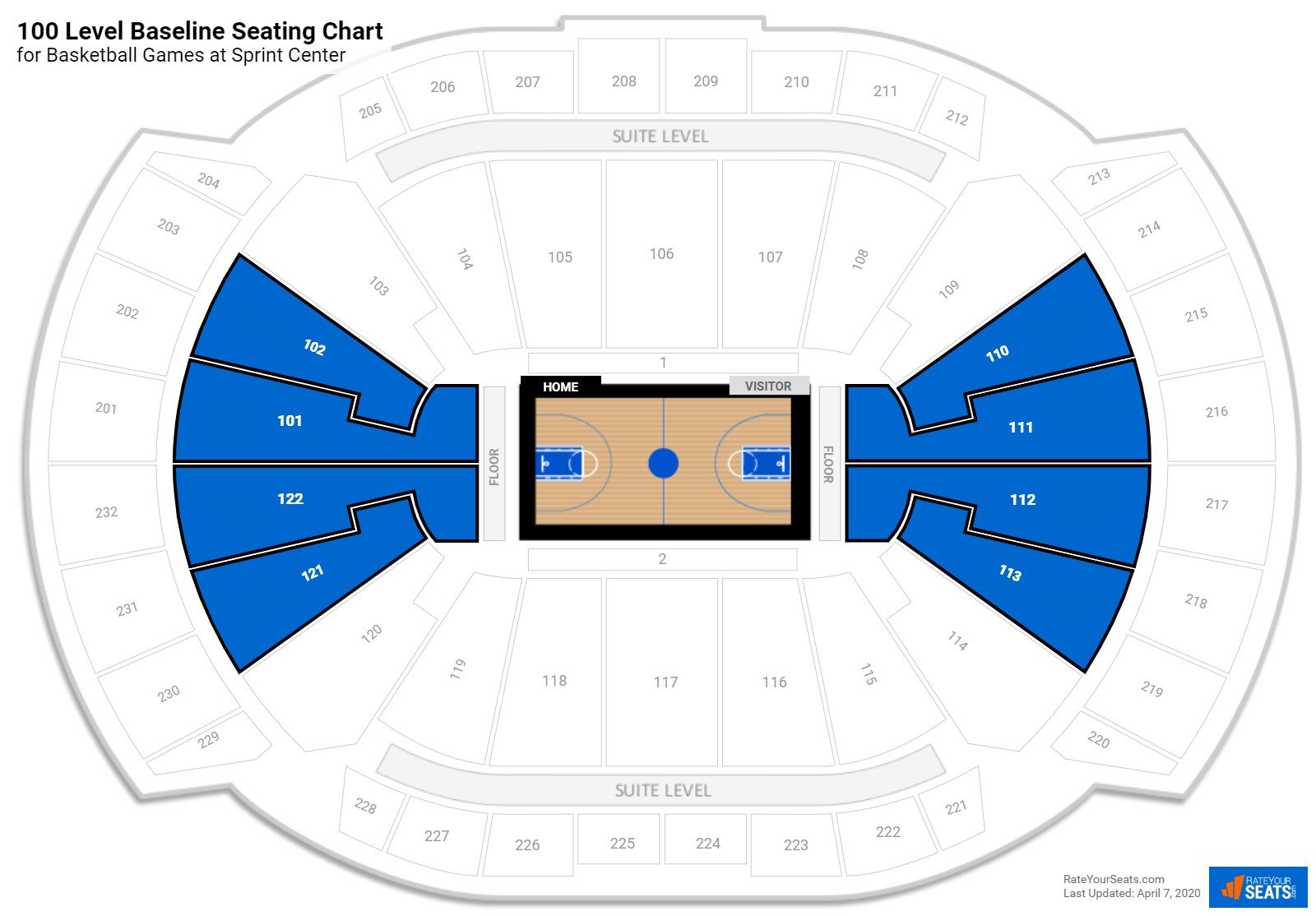This image features a detailed seating chart of the 100-level baseline sections for basketball games at the Sprint Center. The chart highlights a set of prominently large boxes designated for floor seating, suggesting these sections are reserved for owners and VIPs. The basketball court is clearly illustrated, and there is a small blue box indicating the chart was last updated on April 7th, 2020. Another small box designates the area as having reserved seats. The 100-level, as depicted, appears to offer some of the best and most exclusive seating options available, with additional 100-level seats slightly less accessible to the general public.